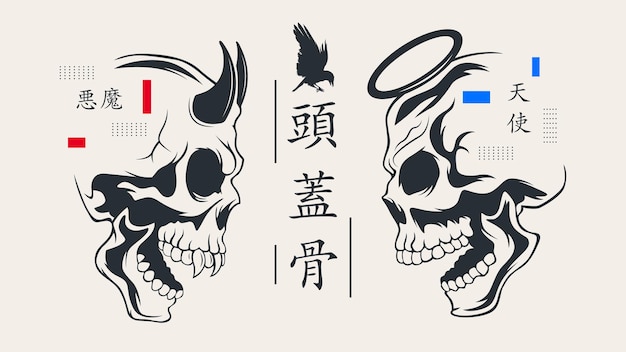The image is a horizontally rectangular, black and white ink vector drawing on a white background. In the center, three Chinese characters are arranged vertically, framed by two bars on each side, creating space between the characters and the surrounding elements. At the top of the first character, a black crow or raven illustration is perched. The focal point features two skulls facing each other from opposing sides. 

The skull on the left, representing a devil, has two black horns on its forehead and fangs in place of its two front teeth. There are also two vertical red rectangles near this skull. On the right, the skull symbolizes an angel, with an angelic halo above its head and a set of normal teeth. Similarly, this skull is accompanied by two blue rectangles. Both skulls feature additional Asian writing near their bases, likely Chinese, Korean, or Japanese characters. The detailed black outlining and intricate designs of the skulls contrast vividly against the white background, emphasizing the strikingly symbolic scene.